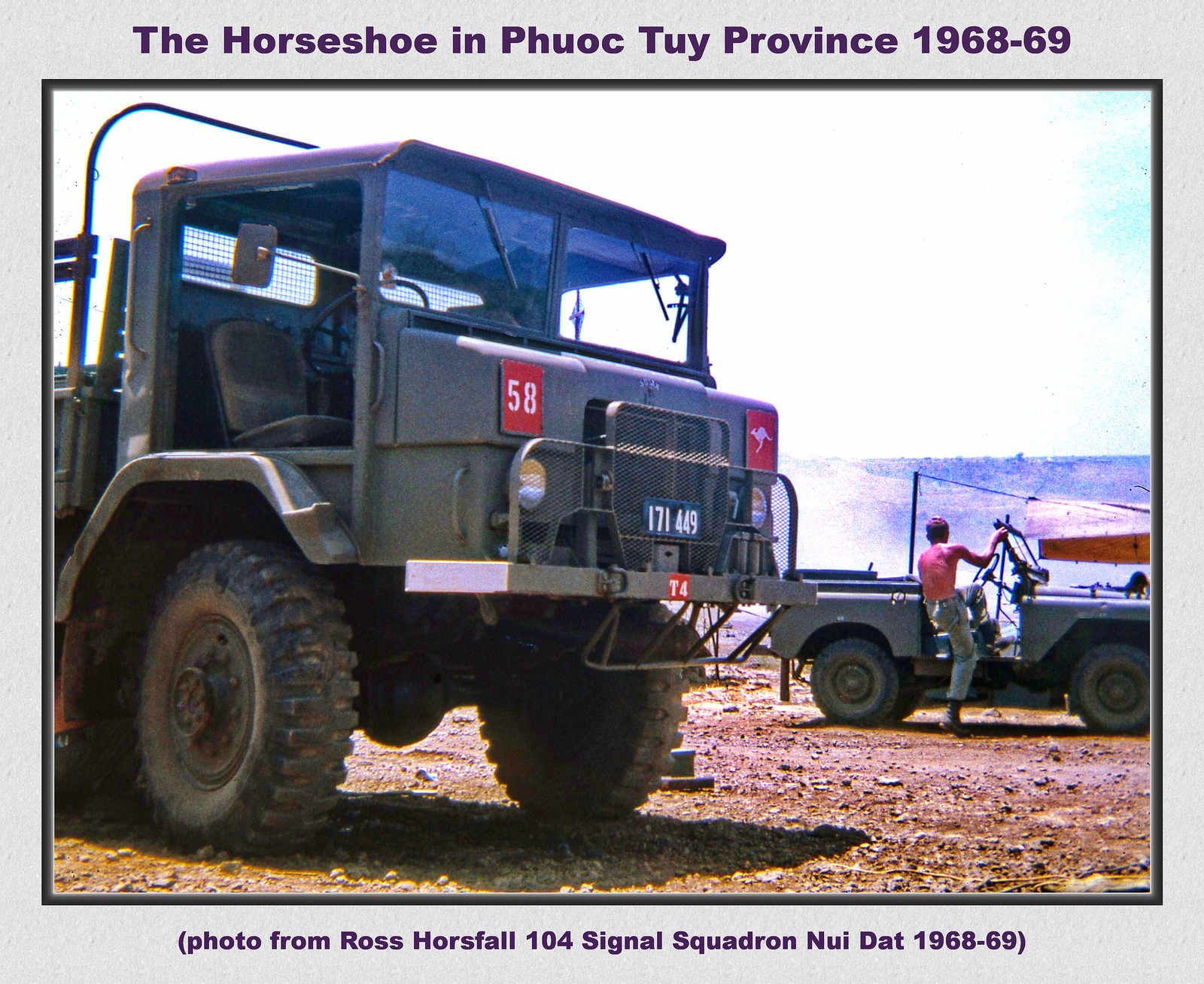This is an image of two military vehicles from the Vietnam War era, specifically taken in Phu Thai Province in 1968-1969. The larger military truck is on the left, painted in army green with distinctive red numbers, red squares, and a kangaroo symbol on its front, along with the license plate 171449 and T4 below it. This truck, possibly used for off-road purposes, has no doors and is equipped with off-road tires, situated on what appears to be muddy ground that could also resemble a beach. Next to it, on the right, is a smaller army jeep, also lacking doors and painted in the same army green. A bare-chested man dressed in army pants is seen actively getting into the jeep, with one leg inside the vehicle and the other still on the ground. The backdrop includes blue skies and gives a sense of being in a foreign, likely war-torn, outdoor environment. Above the image, a caption reads: "The Horseshoe in Phu Thai Province, 1968-1969." Below, another caption states: "Photo from Ross Horsfall, 104 Signal Squadron, Nui Dat, 1968-1969."